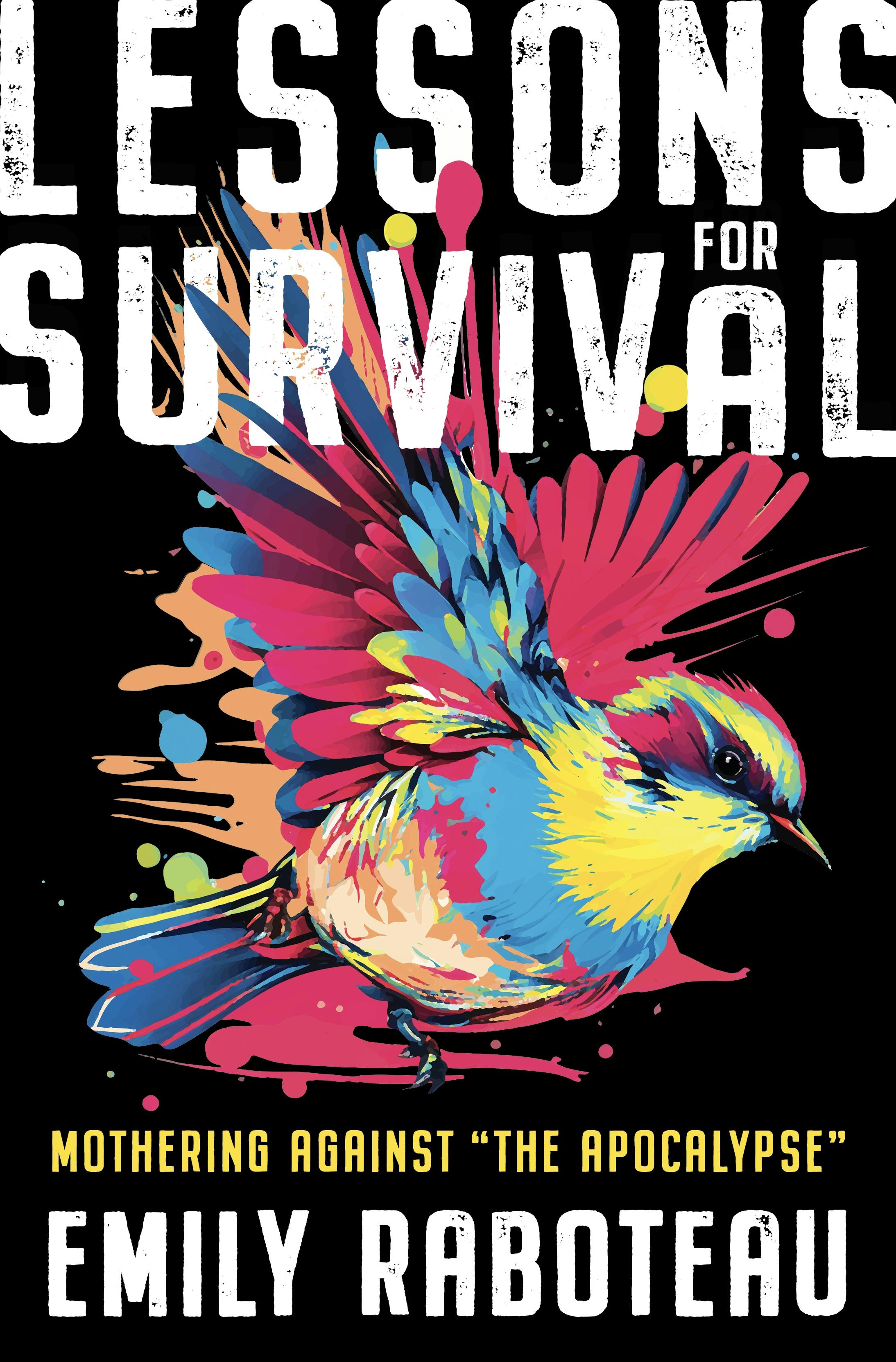This image is the cover of a book titled "Lessons for Survival." Set against a solid black background, the cover features the title in prominent white letters at the top. The focal point is a vibrant, colorful bird positioned prominently in the center. This bird's feathers display a stunning array of colors including bright pink, blue, yellow, and peach, with notable splashes around its figure. The bird has a predominantly blue and yellow body, with black feet, and a head adorned with yellow and blue stripes. Its beak is a mix of pink and yellow, and its eyes are black. Directly beneath the bird, in yellow letters, is the subtitle "Mothering Against 'the Apocalypse'," which suggests a non-fiction theme. Below this subtitle, the author’s name, Emily Raboteau, is displayed in large white letters. The cover beautifully integrates the striking artwork with the thematic elements of survival and resilience.